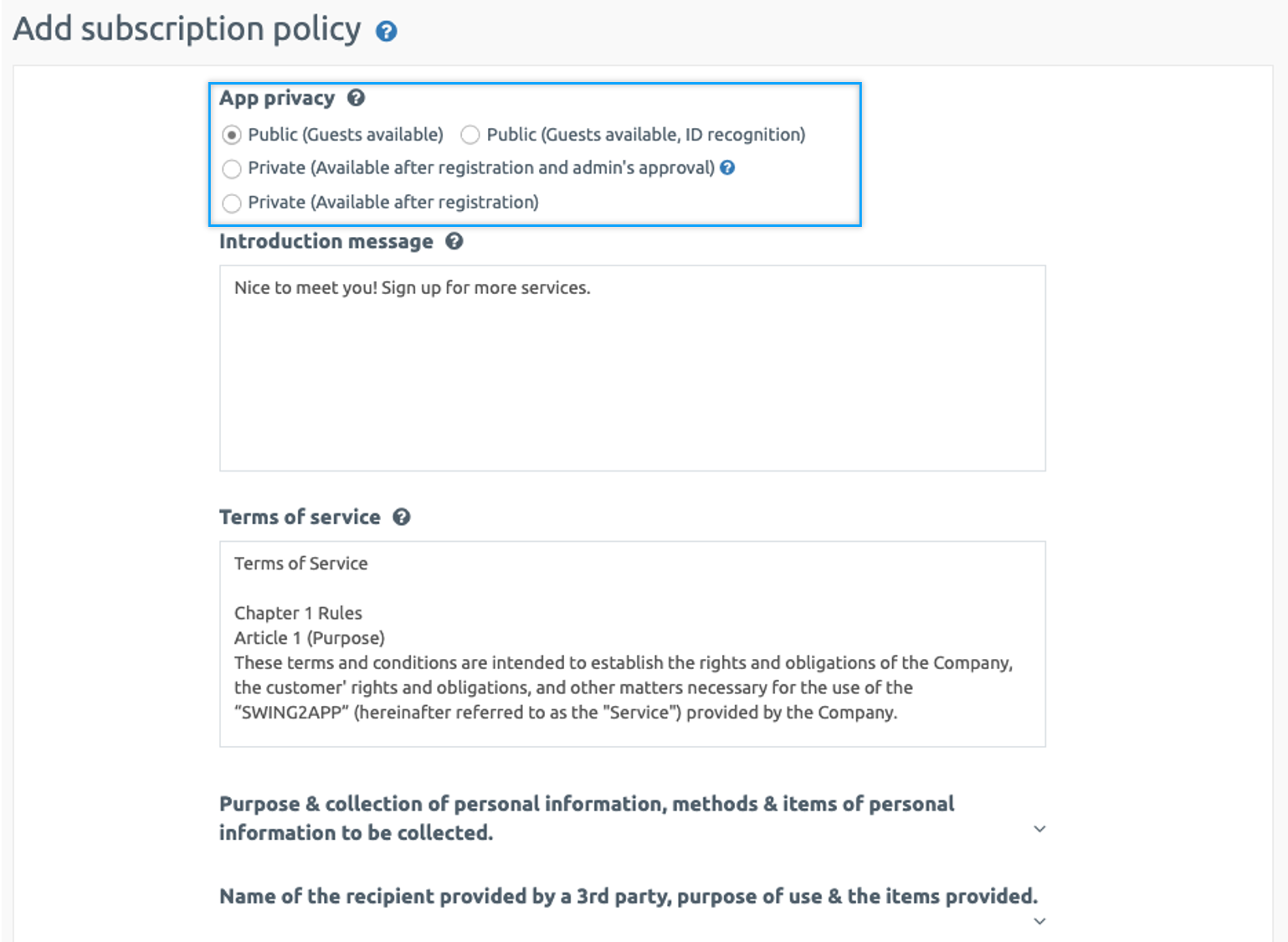This image showcases a detailed screenshot with various informational sections in gray text against the upper left corner. Encased in a light blue bordered box, the first section is titled 'Add Subscription Policy,' followed by 'App Privacy.' The captions for 'Public Guest Availability' and 'Public Guest Available ID Recognition' are also displayed. An additional note mentions that 'Private Access' is available only after registration and administrator approval.

Below this, the screenshot reveals an 'Introduction Message' field featuring a sizable text box containing the greeting, "Nice to meet you. Sign up for more services." Directly under this is a subheading labeled 'Terms of Service.' Under 'Section One - Rules,' it begins with 'Article One – Purpose,' explaining that the terms and conditions aim to define the rights and obligations of both the company and the customers, as well as other necessary information for utilizing the 'Swing to App' platform. Further details listed include 'Purpose and Collection of Personal Information,' 'Methods and Items of Personal Information to be Collected,' and 'Name of the Recipient Provided by a Third Party.' Additionally, it describes the 'Purpose of Use and the Items Provided.'